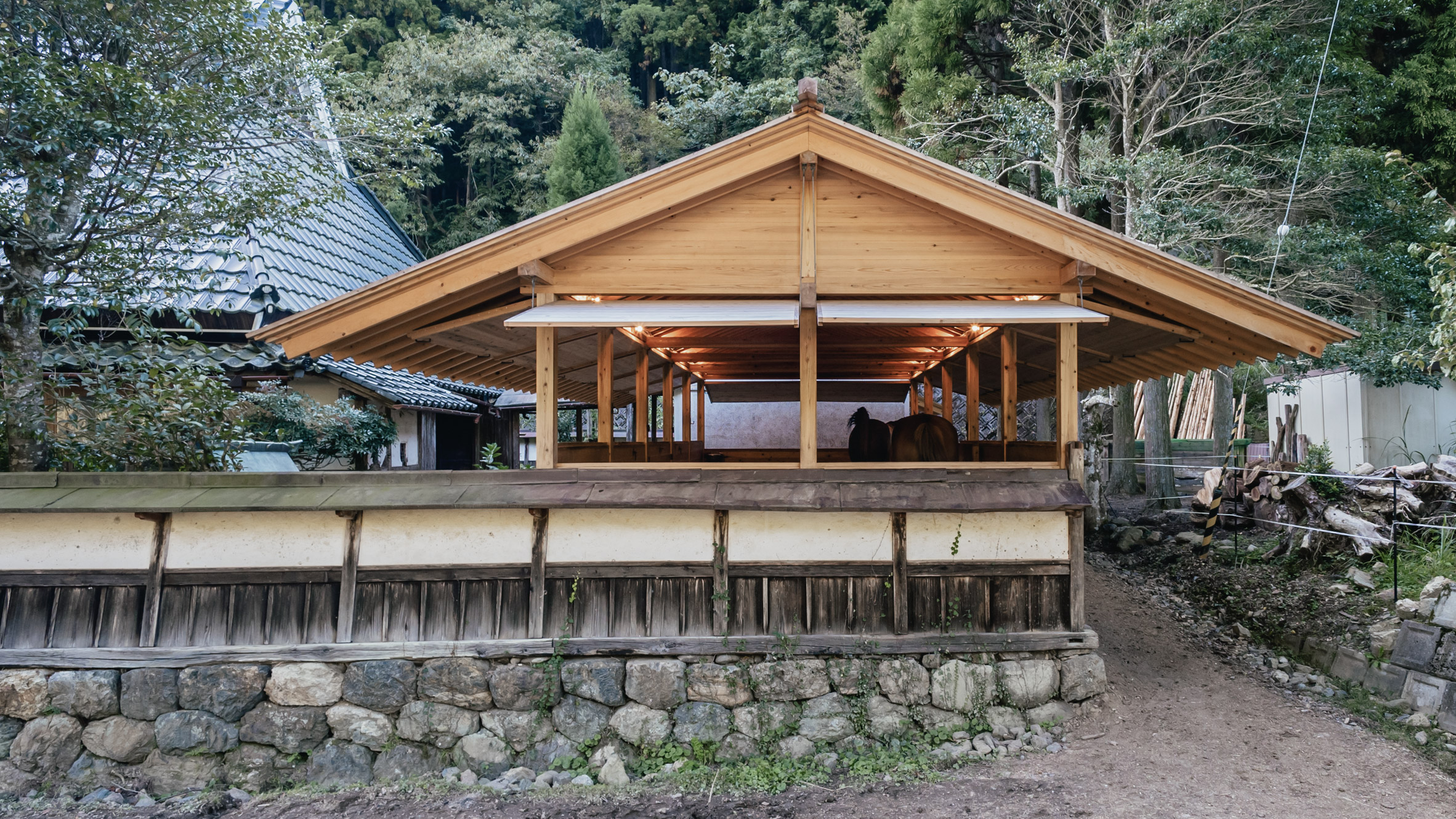This daytime photo captures an outdoor area surrounded by various green and bare trees. The central focus is a covered patio with an A-frame roof supported by light-stained wooden pillars. The sides of the patio are open, and though it's difficult to see inside clearly, there appears to be a human figure and maybe a horse, suggesting it might be a stable. The patio's ceiling reveals rafters, and there are lights hanging from it.

In front of this structure, there's a wall featuring stonework at the bottom topped with a wooden railing. To the left, another building with a tile roof, partly hidden by a tree, is visible. The building's roof tiles are dark green. In the background, a dirt path runs along the right side, bordered by a wire fence that separates the patio area from a pile of chopped wood and a tall, white fence further back. There also seems to be a sign near the pile of wood on the right-hand side. The setting might be a campground or similar outdoor venue.